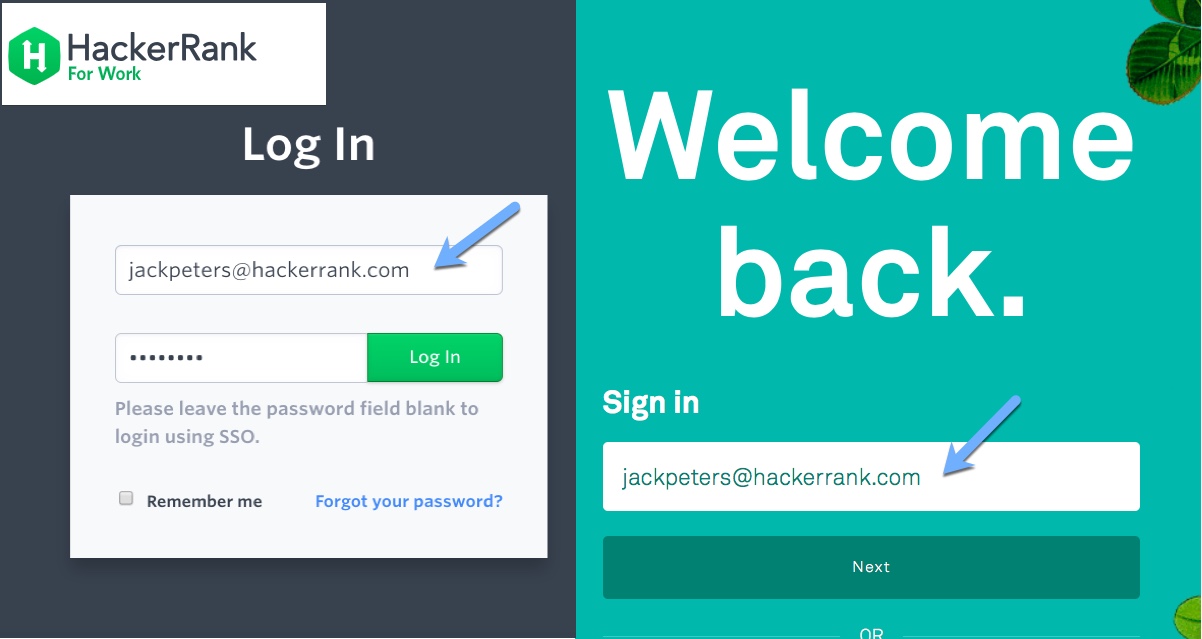The image is a screenshot of a login page for a website. The layout is divided into two sections. The left side features a black background with a white box in the upper left corner, displaying the text "Hacker Rank for Work" in white letters. Below this, there is an icon resembling a circle with flat sides, containing a white "H." Beneath the icon, the word "Login" is prominently displayed in large white letters.

Further down, there is a light gray box with an input field where a website address has been entered. A blue arrow points toward this address. Below this input field, there is another field for entering a password. The "Login" button is highlighted in green. A note underneath instructs users, "Please leave the password field blank to log in using SSO." Additionally, there is a checkbox labeled "Remember me" and a link that says "Forgot your password?" in blue text.

The right side of the image features the text "Welcome back," in large white letters, followed by a period. Below this, it says "Sign in," and an email address has been entered into the input field. Underneath this field, there is a dark green bar with the word "Next," and beneath that, the word "or".

The image appears to be partially cut off, as parts of the design are incomplete. In the upper right corner, there is an image of some leaves, and in the lower right corner, a single lighter green leaf is visible. The website's design is colorful and eye-catching, utilizing a stark contrast between the black background and green accents.